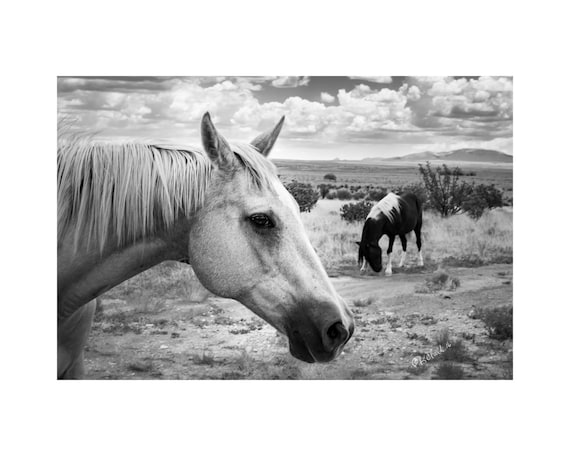In this detailed black-and-white photograph, we see a close-up side view of a large, beautiful white horse with a mane combed over to the side, standing in a dry, flat terrain. Her features, including a white nose with a black tip, black eyes, and erect ears, are prominently visible. Behind her, a black and white horse is grazing, its white upper back and hooves contrasting against its darker body. The landscape around them appears arid, with dry soil and lifeless grass interspersed with desert plants and sagebrush. In the background, a flat expanse leads to distant hills. Puffy gray clouds dominate the sky, with only a few small openings revealing the sky's true shade. The atmosphere is underlined by a sense of dryness and the natural debris scattered across the ground.